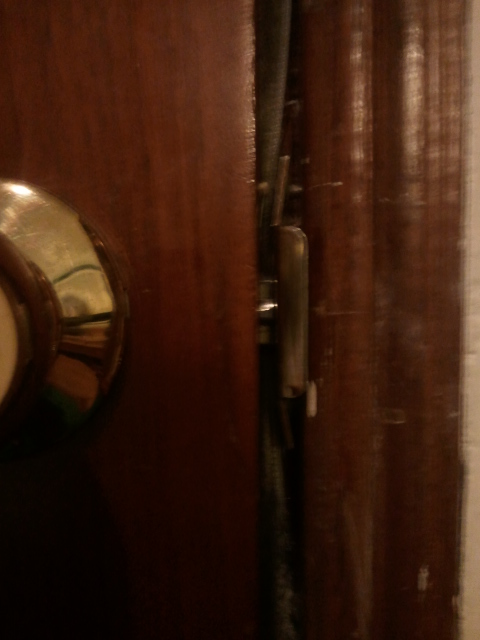This extreme close-up color photograph captures the intricate details of a dark oak wooden door as it begins to open at the latch. Centered and slightly out of frame to the left, a bronze doorknob, mostly cut off, hints at the mechanism used to manipulate the lock. The door, edged towards the right of the image, reveals the door frame and its hardware—a brass catch plate aligning with the door's brass latch. A noticeable gap between the door and the frame highlights the tarnished craftsmanship, with reflective varnished surfaces catching the light towards the top right. The door frame’s right-side strip appears planed away or damaged, contrasting in a lighter beige tone. Some splinters and reflections suggest forced entry, further emphasized by the flash illuminating the door jamb.